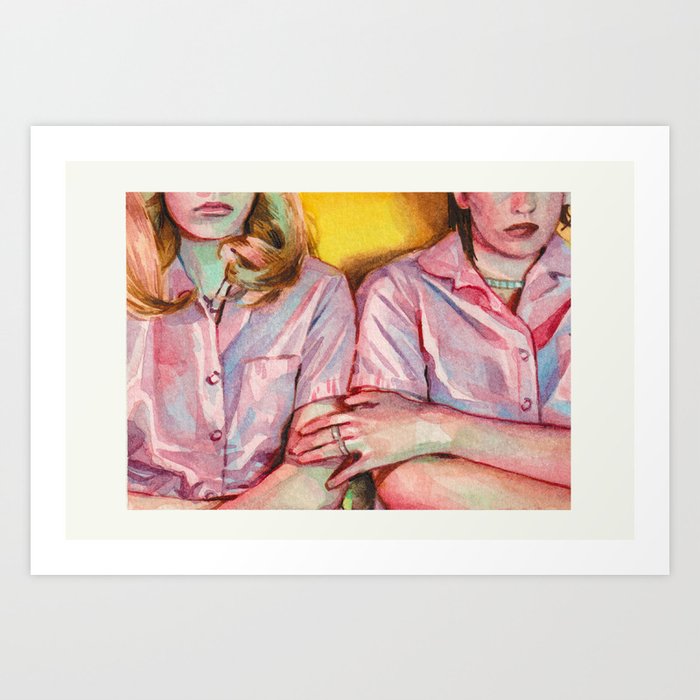This image is a painting, likely done in watercolors, depicting two women seated or standing closely together, with the composition showing only from their noses downward. Their heads are partially out of frame, cutting off above their noses, emphasizing their frowning expressions. The women, one with blonde hair and the other with brown hair, are facing the viewer and appear to be wearing similar or identical short-sleeved blouses in shades of pink, mauve, and blue, suggesting they may be uniforms. The woman on the right is reaching over, gently touching the arm of the woman on the left just above the elbow, and her hand is adorned with two simple rings on the middle and ring fingers. Both women wear necklaces, adding to their coordinated appearance. The painting is set against a yellow background. It is framed with a cream-colored inner border and a white outer frame, and it hangs on a light gray wall.